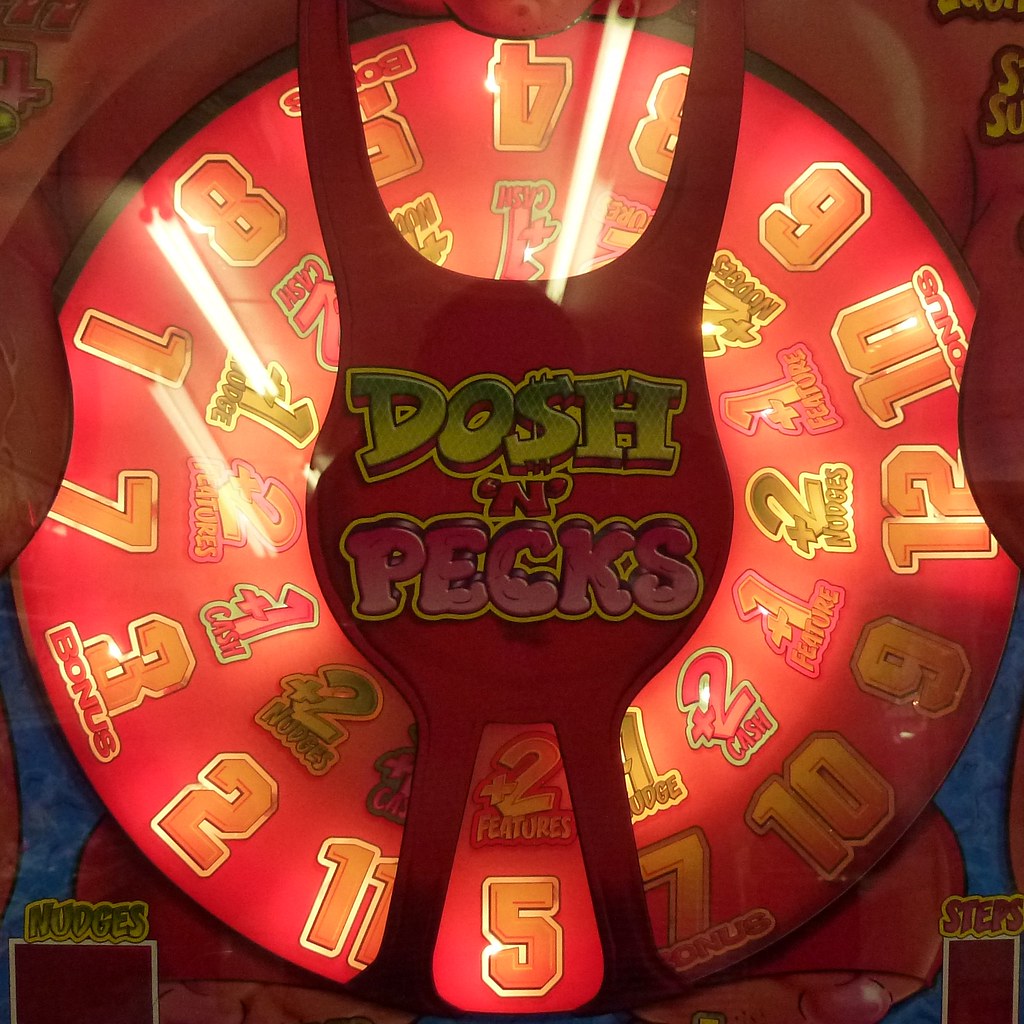This square image showcases a vibrant arcade game, reminiscent of a spin-the-wheel setup. Dominating the frame is a large, circular wheel, whose edges extend to the boundary of the image. The wheel itself stands out with its red illuminated background, and around its outer edge are numbers ranging from 1 to 12, written in orange with a gold border, arranged in a non-sequential order. Moving closer to the center of the wheel, there are a series of smaller numbers, each accompanied by a plus sign or an "X" and some descriptive text beneath them, suggesting potential bonuses or features such as "plus two cash" and "plus one feature." The wheel is crowned by a red metallic portion, adorned with graffiti-like text in green and pink, spelling out "Dosh ‘n’ Pex," with "Dosh" characterized by a green dollar-esque 'S' and "Pex" styled to appear muscular. The image further details areas indicating game statuses, such as 'nudges' in the bottom left corner and 'steps' on the right side, emphasizing the game's complex and interactive features.